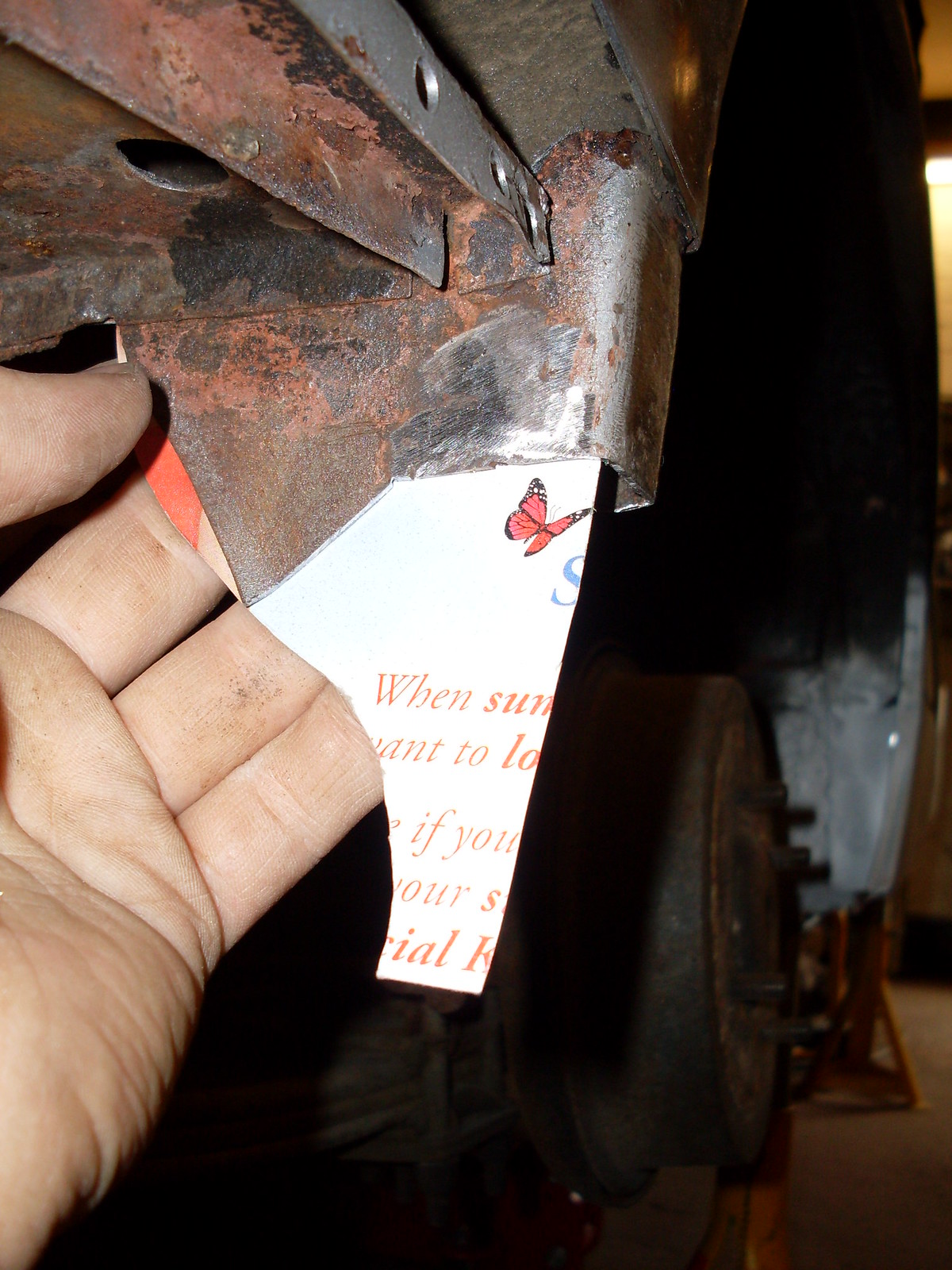This full-color photograph, taken at night, captures a close-up view of a Caucasian hand holding a torn piece of paper against a mysterious metal device that appears to be rusted. The piece of paper, which is notably damaged, features a red, black, and white butterfly in its upper corner and a blue "S" beneath the butterfly. The paper is fragmented but bears some legible text that includes phrases like "when sun to yours." Dirty hands and a brown ground, possibly with chairs, are faintly visible in the background, adding to the complexity and obscurity of the scene. The purpose of the metal device remains unclear, though it has a peculiar shape that hints at some functionality perhaps related to shredding or cutting. The extreme close-up framing makes it challenging to discern the complete context or actions taking place in the image.